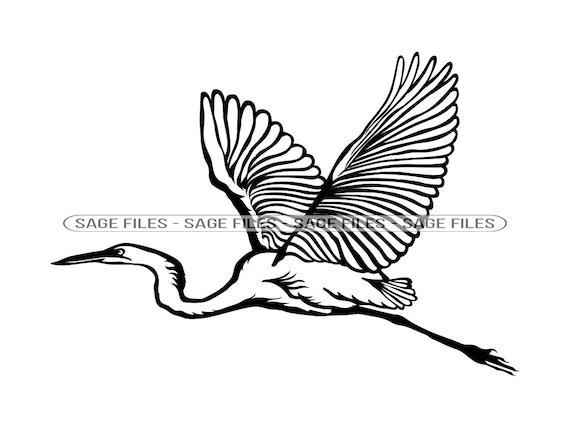The image features a flying bird, likely a crane or heron, positioned against a plain white background with no visible borders. The bird, approximately three to four inches wide from the tip of its beak to the tip of its feet and about two inches high, is flying towards the left. It has a long, straight, thin beak, a narrow head, and a neck that curves gently down and extends back. The wings are extended upwards in a V-shape. The bird's long black legs trail behind it. Overlaying the image, there is a semi-transparent watermark that reads "SAGE FILES," repeated four times, each phrase separated by a dash. The design is composed of black lines, giving it a silhouette-like appearance, similar to a minimalist tattoo or a graphic design work.